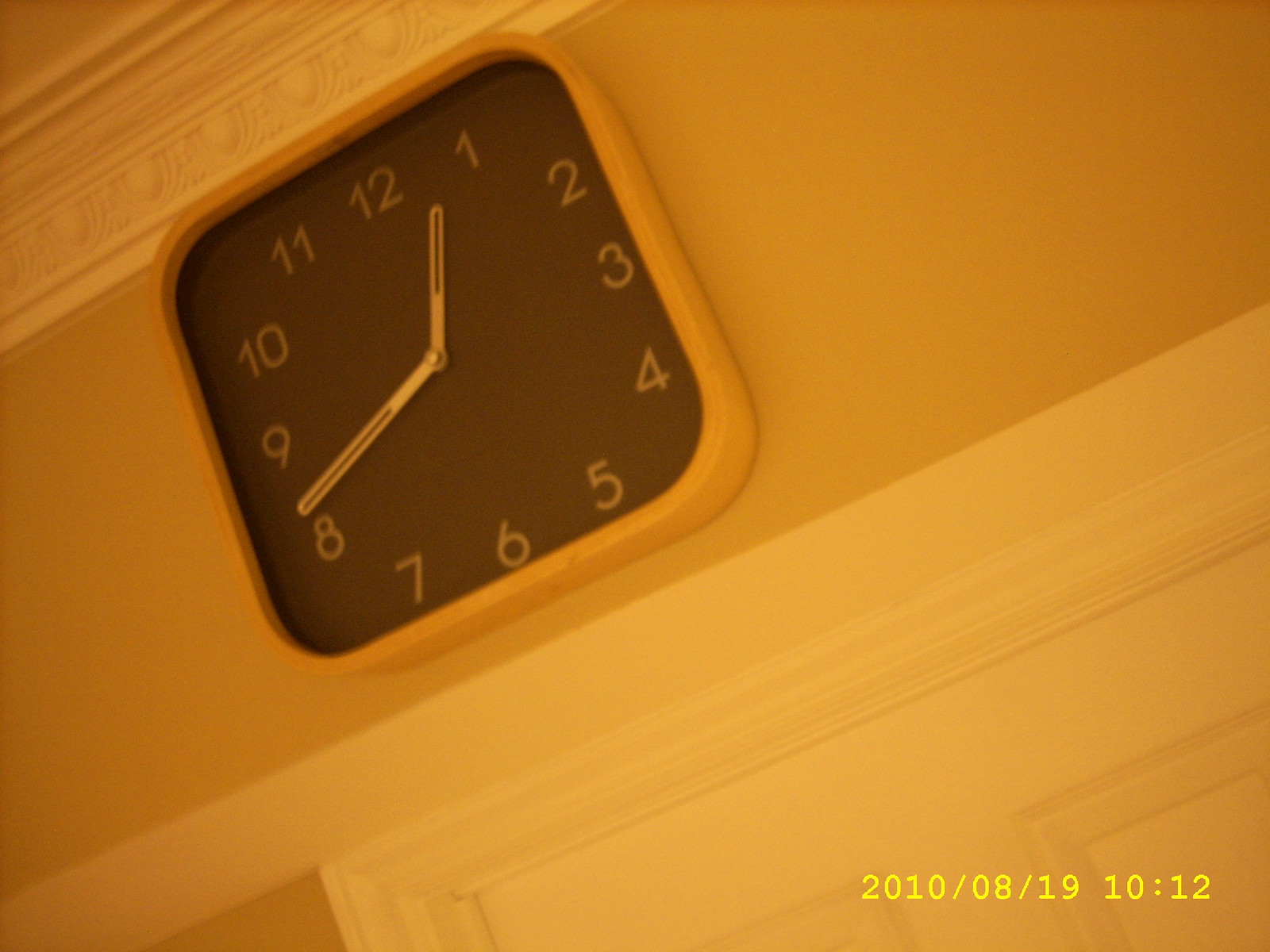This photograph captures a slightly tilted image of a square-shaped wall clock mounted just below decorative trim on a wooden wall, positioned above a white door with white framing. The clock has an off-white, yellowish background and a brown face featuring traditional numbers from 1 to 12, clearly printed in white or brownish lettering. The clock's hands, which indicate the time as approximately 12:42, are white with brown stripes. Above the clock, a textured ledge or decorative trim is visible. The entire image has a yellow tint, and in the bottom right corner, a yellow timestamp reads "2010/08/19, 10:12."